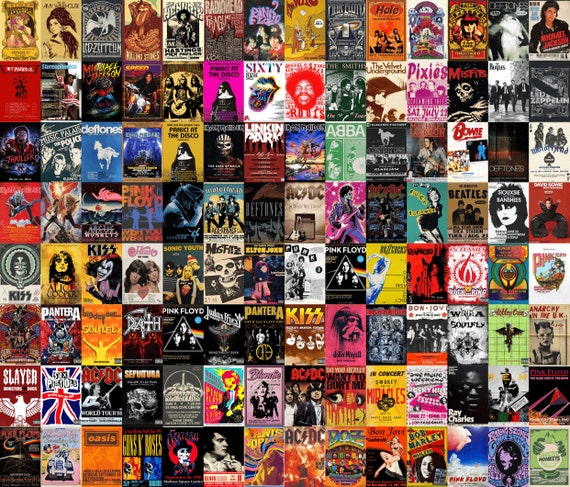The image is a meticulously crafted collage of numerous iconic album covers arranged in a grid-like fashion, predominantly featuring rectangular shapes. It vividly presents a spectrum of vivid colors, mainly yellow, red, pink, white, blue, green, and orange, creating a visually striking tapestry. Among the celebrated artists, the collage showcases timeless figures such as Amy Winehouse, Michael Jackson, and Elvis Presley, along with bands like KISS, ACDC, and The Beatles. The eclectic mix spans multiple genres, from metal to pop to rock, representing both contemporary and retro music.

The grid features well-known albums from artists like Bob Marley, Pink Floyd, Guns N' Roses, Oasis, Motley Crue, Steppenwolf, Slayer, Pantera, Deftones, Linkin Park, and The Misfits. This visually dense artwork is composed of several, some repetitive, album covers identifiable by their iconic imagery, though the small size makes some harder to discern. Notable album covers include Guns N' Roses' "Use Your Illusion 1 and 2," multiple appearances by ACDC and KISS, as well as standout pieces by Michael Jackson, Jimi Hendrix, and Elvis Presley.

This collage comes across as a celebration of musical history, piecing together legendary acts and albums into a cohesive and colorful homage to music's vibrant evolution.